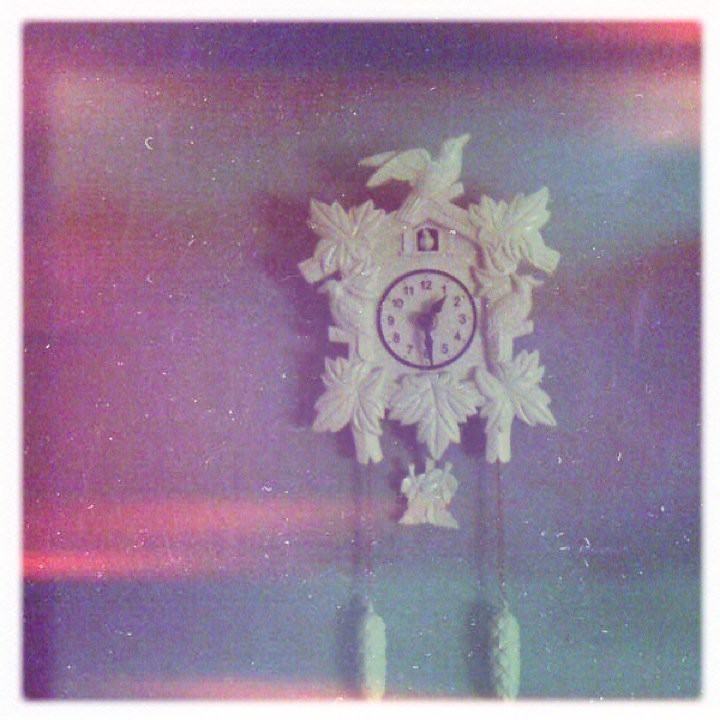The image depicts a charming white cuckoo clock mounted on a multicolored wall featuring shades of purple, blue, and pink. Due to the low quality of the picture, the wall appears to have various colors blending together. The clock itself is beautifully detailed, designed to resemble a little house adorned with intricate leaves and birds. The clock casing and decorative elements, including the leaves and birds, are made of white plastic. Prominently, a large white bird, appearing to take flight, perches atop the clock. The central clock face is white, encircled by a black rim, with black numerals and hands marking the hours. Just below the top, a small door reveals a tiny cuckoo bird, emphasizing its function as a cuckoo clock. At the bottom, two chains dangle down, each ending in a long white weight, completing the elegant and whimsical design of this wall-mounted timepiece.